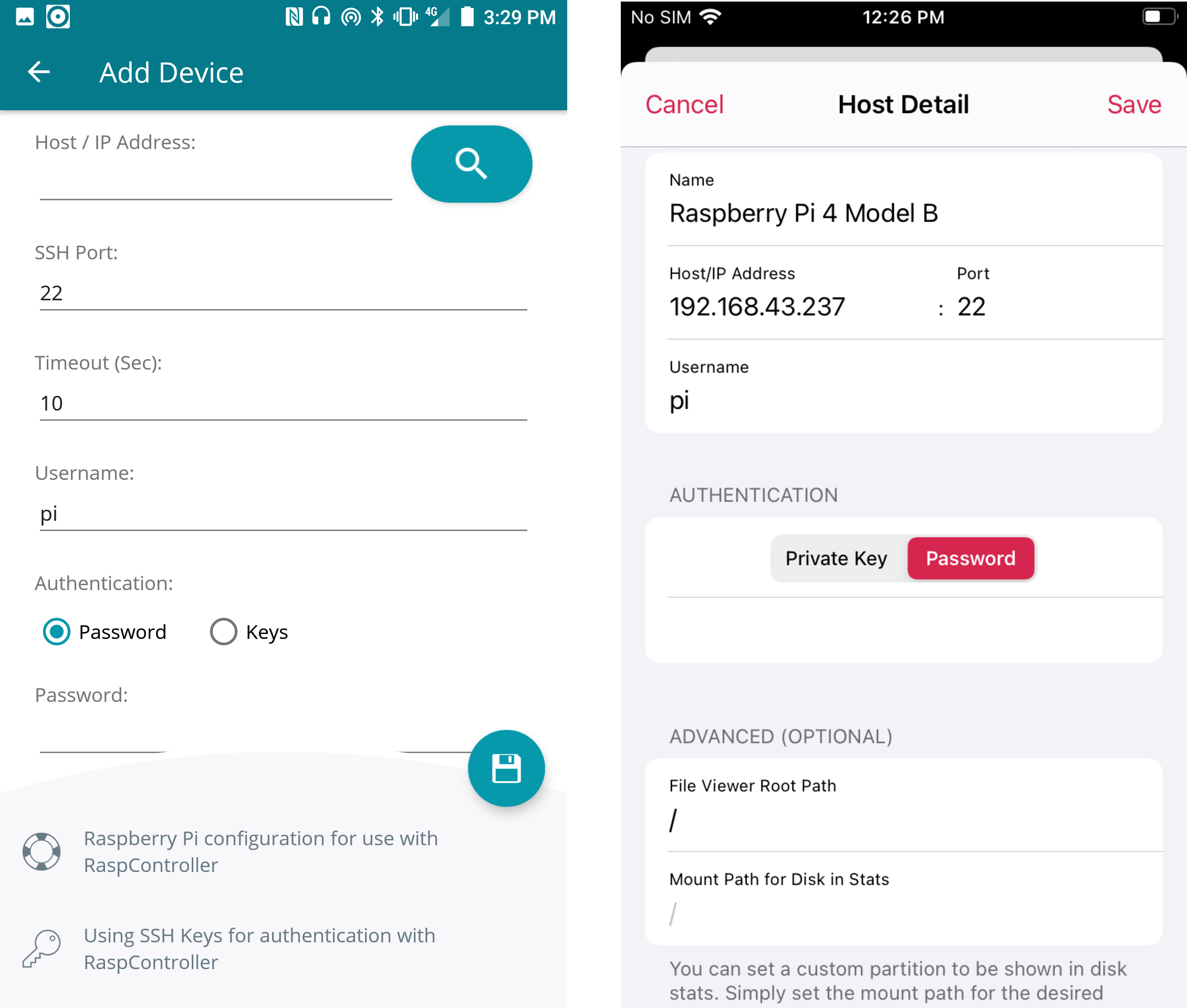### Caption:
The image features two smartphone screenshots detailing the configuration settings for a Raspberry Pi using the RASP controller app. 

#### Left Screenshot:
The screenshot showcases an interface with various top icons, including Bluetooth, battery, and 4G signal indicators. The header is highlighted in blue, displaying the text "Add Device" in white. Below, several fields are present:
- **Host**: IP address 
- **SSH Port**
- **Timeout**
- **Username**
- **Authentication**: Set to "password" with an alternative option for "keys."

At the bottom, gray text reads, "Raspberry Pi configuration for use with RASP controller," followed by a line stating, "Using SSH keys for authentication with RASP controller."

#### Right Screenshot:
The second screenshot indicates "No SIM" with a Wi-Fi symbol and shows the time as 12:26 p.m. along with a battery indicator. It includes action buttons labeled "Cancel," "Host Detail," and "Save." The configuration details for a Raspberry Pi 4 Model B are as follows:
- **Host/IP Address**: 192.168.43.237
- **Port**: 22
- **Username**: pi
- **Authentication**: Set to "password" with an option for a private key.

In the "Advanced" section, labeled as optional, there are settings for a "File Viewer Root Path" and a "Mount Path for Disk Stats." It mentions the ability to set a custom partition to be displayed in disk status and adjust the mount path as desired.

The detailed text concludes abruptly with the phrase "you can actually set the mount path for the desired."